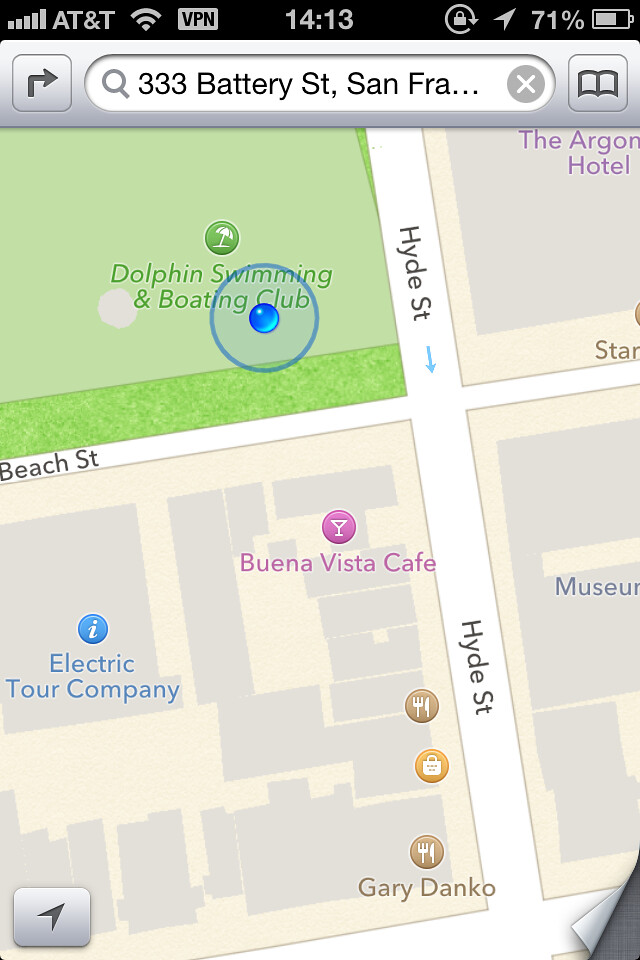The screenshot appears to be taken from Google or Apple Maps on a smartphone or an iPad. At the top of the screen, typical device symbols are visible: AT&T with a Wi-Fi signal, the time marked as 14:13, and the battery level at 71%. In the search bar, the address "333 Battery Street, San Francisco" is partially visible. The map focuses on the intersection of Hyde Street and Beach Street, pinpointing the Dolphin Swimming and Boating Club. Nearby landmarks include the Buena Vista Cafe, Electric Tour Company, Gary Danko restaurant, a museum, and the Argonne Hotel.